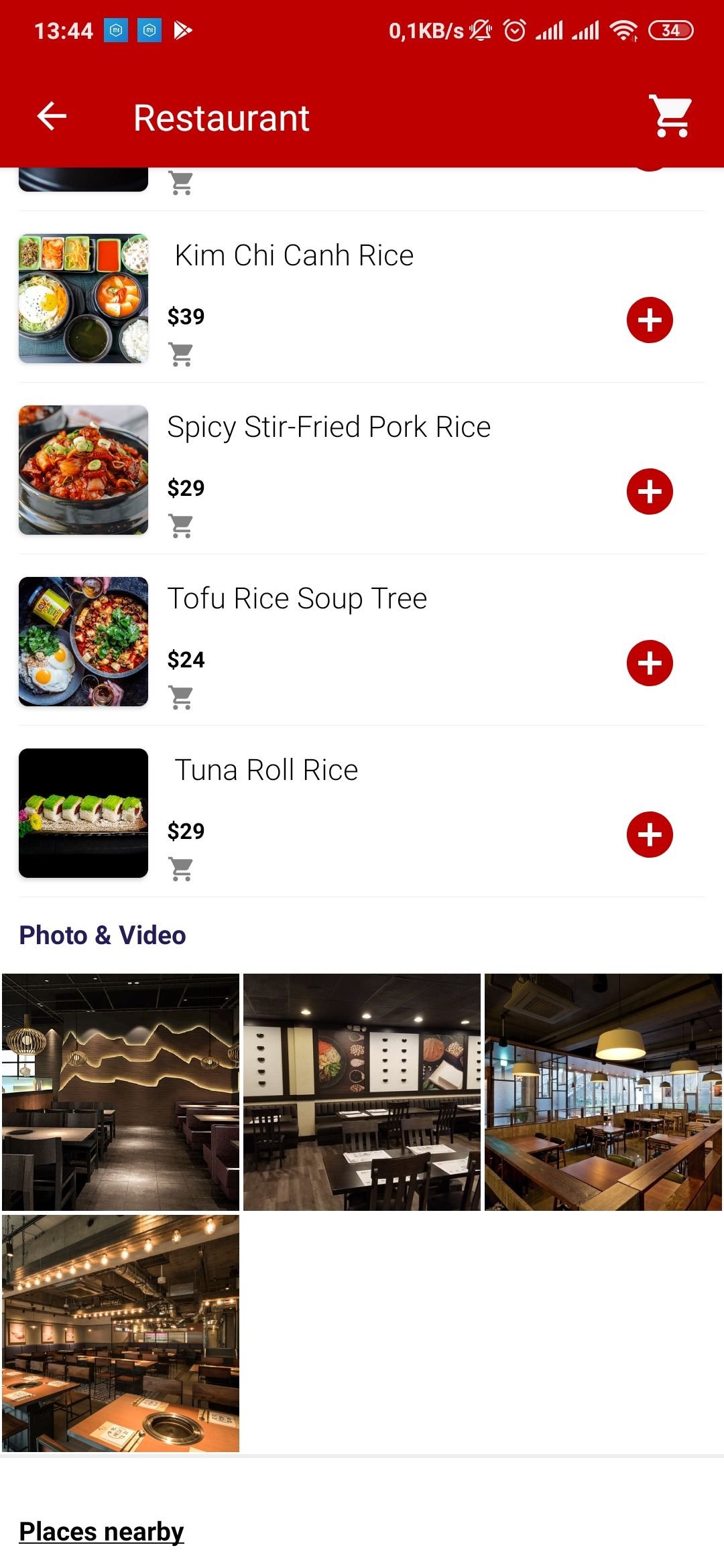The image features a digital food ordering interface. At the top of the screen, a red box displays the time as 13:44 with four bars of signal strength and an arrow pointing left labeled "restaurant." There is also a shopping cart icon nearby. 

Beneath the red box, the interface presents a menu on a white background. The left side of the screen displays thumbnail photos of various food dishes, with each photo accompanied by the name of the dish, its price in the center, and an "Add" button on the right side. The "Add" button is red with a plus sign in the middle.

The menu lists the following dishes:
- Kimchi Con Rice priced at $9.39
- Spicy Stir-Fried Pork Rice priced at $29
- Tofu Rice Soup priced at $24
- Tuna Roll Rice priced at $29

Below the menu, there is a section labeled "Photo and Video," showcasing four pictures of the restaurant's interior. These photos highlight the tables and light fixtures on the ceiling. Lastly, there is text indicating "Place It Nearby" under the image section.